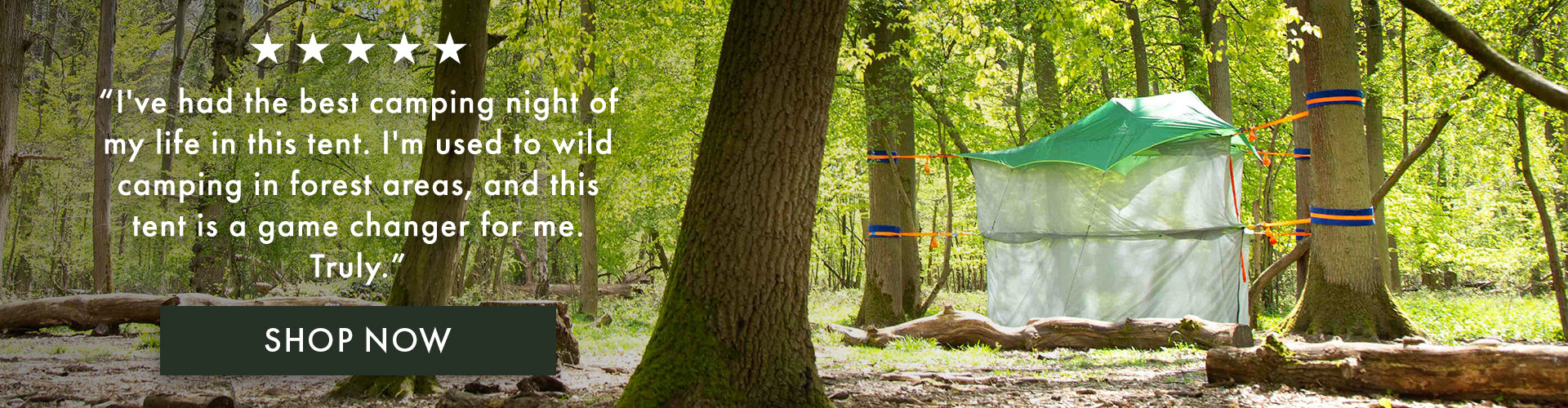The image is a horizontally oriented advertisement set in a woodsy, forested area with a sandy ground. On the left side, the ad features a review comprising five white stars followed by a testimonial in white text spread over four lines. The review reads: "I've had the best camping night of my life in this tent. I'm used to wild camping in forest areas and this tent is a game changer for me, truly." Beneath the review is a thin gray rectangle with the words "shop now" in white, indicating a call to action. The rest of the image showcases a forest scene with various tree trunks extending off the top of the image. To the right of the "shop now" sign, a prominent tree trunk diagonally ascends, while additional trees stand further right.

In the middle and background of the image, a unique tent-like structure is visible. The tent features gauzy, white walls and a green tarp roof, supported between three trees. Orange and blue ropes secure the tent to the trees. In the foreground, to the bottom right corner, a log is lying on the ground, extending diagonally from the bottom right toward the left. The entire scene is framed by a dense backdrop of more incomplete trees, cementing the outdoor, forest atmosphere of the setting.